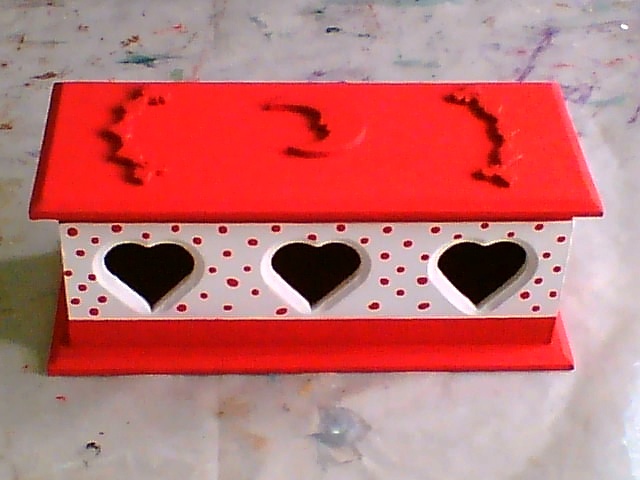In the photograph, a small red and white box is placed on a smooth, white epoxy table featuring a swirl of vibrant colors including purple and blue splotches. The box, possibly made from wood or a wood composite, displays intricate detailing: its bottom third is painted red, transitioning into a white section adorned with red polka dots. The front face of the box has three heart-shaped cutouts. The red lid is decorated with three flat, painted red shapes, including a crescent moon in the center. The box appears to sit on parchment paper atop the table, adding a touch of rustic charm to the overall scene.